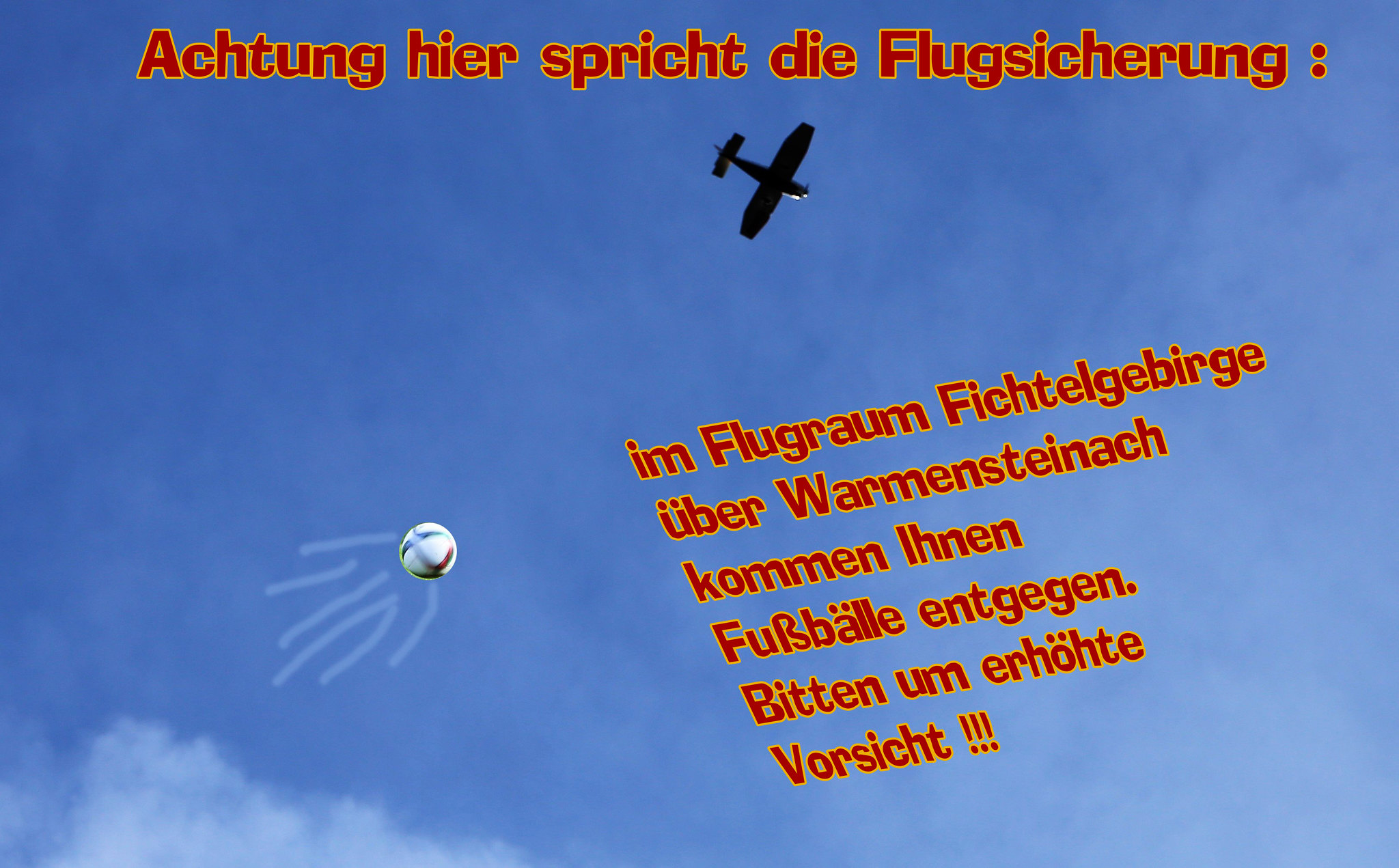The photograph captures a vibrant blue sky adorned with wispy white clouds, predominantly situated in the bottom left and central portions. Centered in the upper portion of the image is a black biplane or single-engine aircraft, possibly a Cessna or Piper, appearing as a silhouette flying from the top left to the bottom right. The plane's full outline, including the wings, fuselage, tail fin, and front engine, is clearly discernible. Superimposed in the bottom left corner is an edited image of a soccer ball, adorned with white to gray motion lines that give the illusion of the ball being kicked towards the airplane. The ball features a playful design with eyes and a smile. The image is overlaid with German text in a distinct red font with an orangish-yellow border, located at the top and along the bottom right third of the photograph. The text reads "Achtung, hier spricht die Fliegerstrahlung" ("Attention, this is the aircraft radiation speaking"), followed by additional lines in German, presumably describing the plane. The overall bright, sunny day enhances the cartoonish and animated effect of the composition.